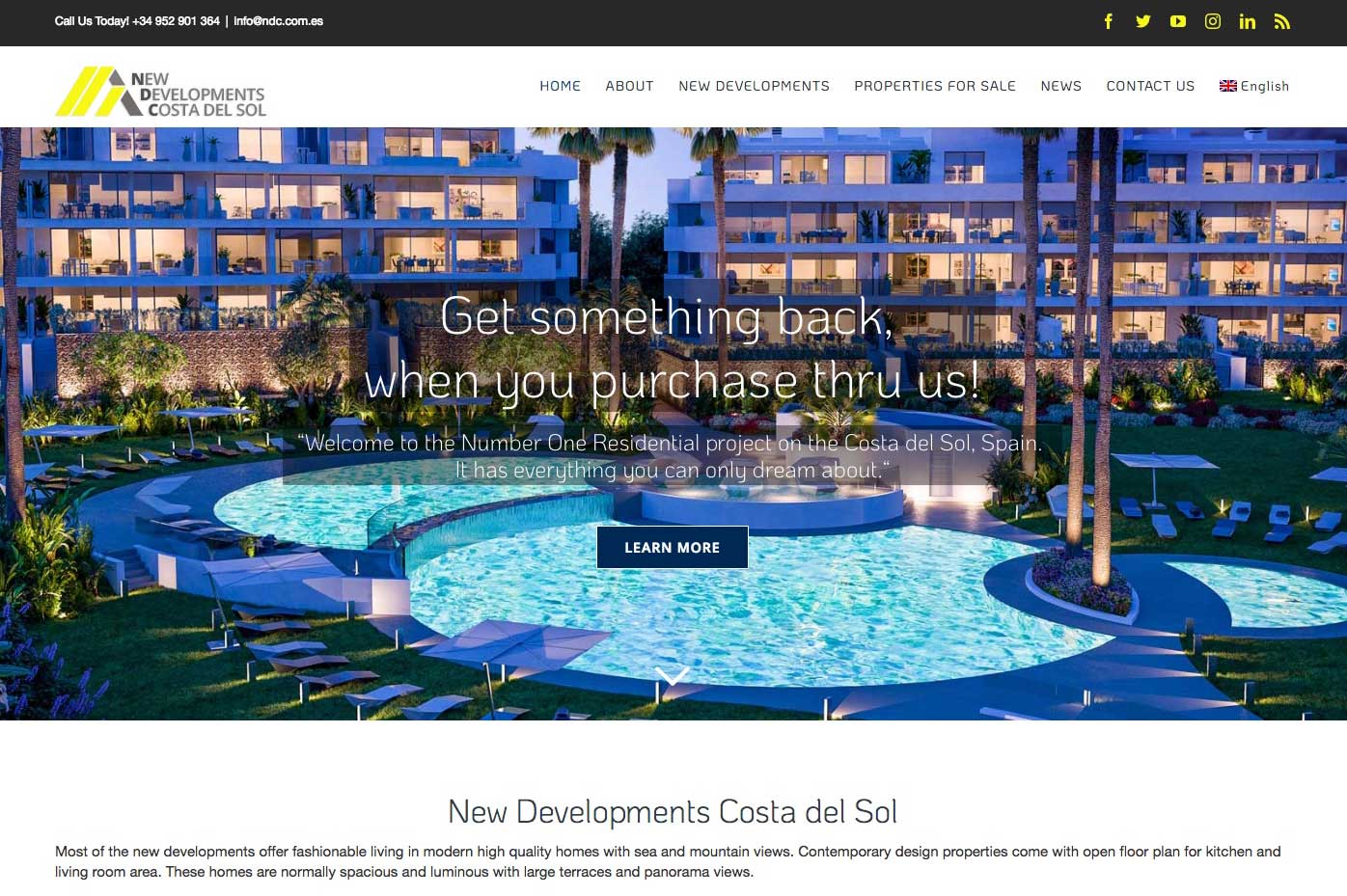**Homepage of New Developments Costa del Sol: A Glimpse into Modern Living**

At the top of the homepage, a prominent banner encourages visitors to "Call Us Today" with the contact number +34 952 901 364 and an email address info@ndc.com. The site prominently features logos for social media platforms including Facebook, Twitter, YouTube, Instagram, LinkedIn, and a Wi-Fi icon.

Below the banner, the New Developments Costa del Sol logo is displayed in a white box. This logo consists of three arches, where two are triangular and of the same size, and the third is slightly smaller. Next to the logo, a navigation menu offers links to Home, About, New Developments, Properties for Sale, News, and Contact Us, along with a language option indicated by the flag of Great Britain.

The main image on the homepage presents a stunning scene of a luxurious residential complex rather than a hotel resort. The scene captures three illuminated pools surrounded by deck chairs, a beautifully maintained lawn, and tall palm trees. The buildings boast open balconies, offering a glimpse into the elegantly designed interiors. The image is set at dusk, enhancing the ambiance with soft, serene lighting.

Below the captivating image, a prominent text section reads:
"New Developments Costa del Sol: Most of the new developments offer fashionable living in modern high-quality homes with sea and mountain views. Contemporary design properties come with an open floor plan for the kitchen and living room areas. These homes are normally spacious and luminous, with large terraces and panoramic views." 

This detailed description highlights that these are indeed homes designed for modern, luxurious living, providing all necessary information for potential residents.